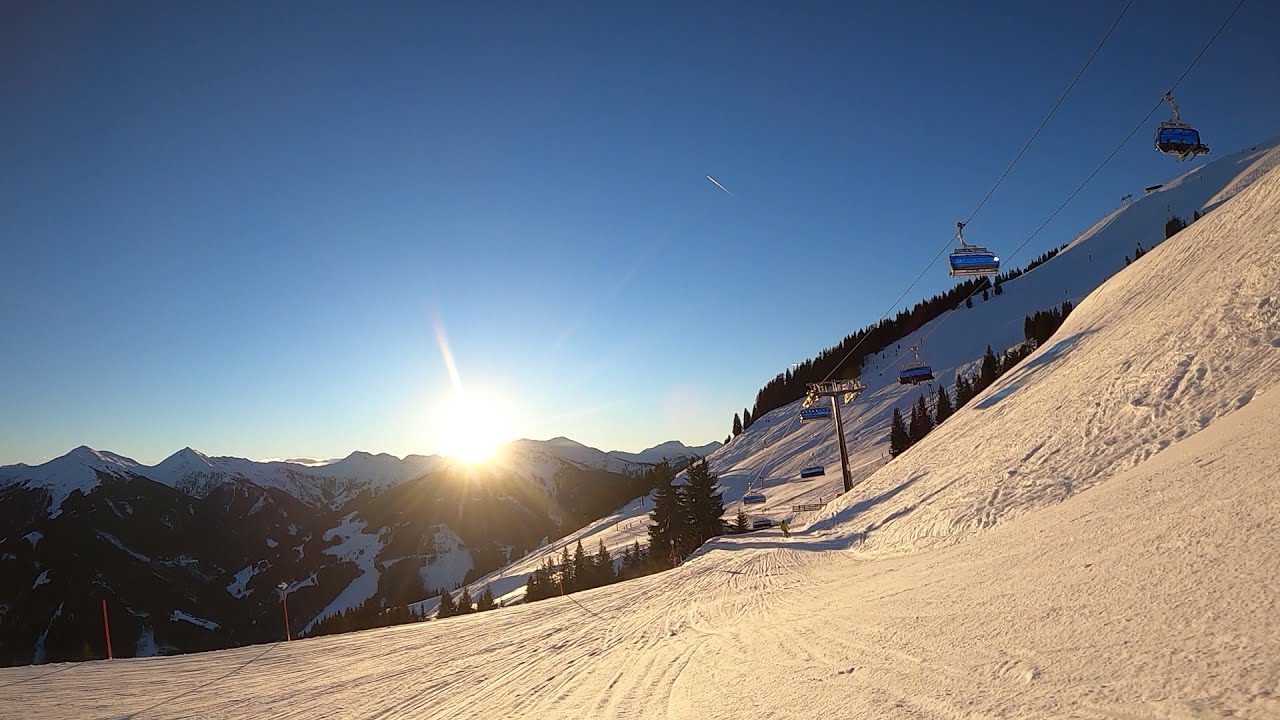In this captivating photograph of a snow-covered ski resort, the scene is dominated by a beautiful sunset, setting the sky ablaze with warm hues. The sun is positioned just left of center, casting a golden glow over the entire landscape. Snow-blanketed mountains stretch from the bottom left, running through the center, and meet the horizon where the sun dips behind them. The serene, clear blue sky is largely unblemished save for a distant plane's contrail.

To the right side of the image, a ski lift with blue-backed gondolas ascends and descends the slope, which is also on the right. The slope is dotted with various ski tracks, evidence of recent skiing activity. Evergreen trees are scattered throughout the center and towards the right, adding a natural green contrast to the snowy white terrain. Distant, snow-capped peaks are visible, enhancing the sense of expansive wilderness. No skiers are in immediate view, leaving the viewer to appreciate the untouched beauty of the scene.